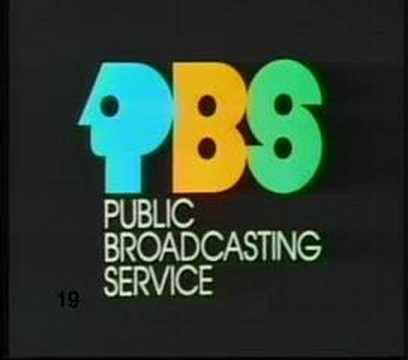The image is a simple yet striking poster for PBS, set against a completely black square background. Dominating the center, the colorful PBS logo features three stylized bubble letters: a neon blue "P" that doubles as the silhouette of a face with a small circular eye, an orange "B" with two circular holes, and a green "S" also featuring two circular holes. Below these vibrant letters, the full name "PUBLIC BROADCASTING SERVICE" appears in all capital, white sans serif font, aligned to the left and stacked on three separate lines. On the left-hand side at the bottom of the image, the number "19" is subtly displayed, adding a touch of asymmetry to the overall composition. The combination of the bright neon letters and the stark black background creates a visually striking design.